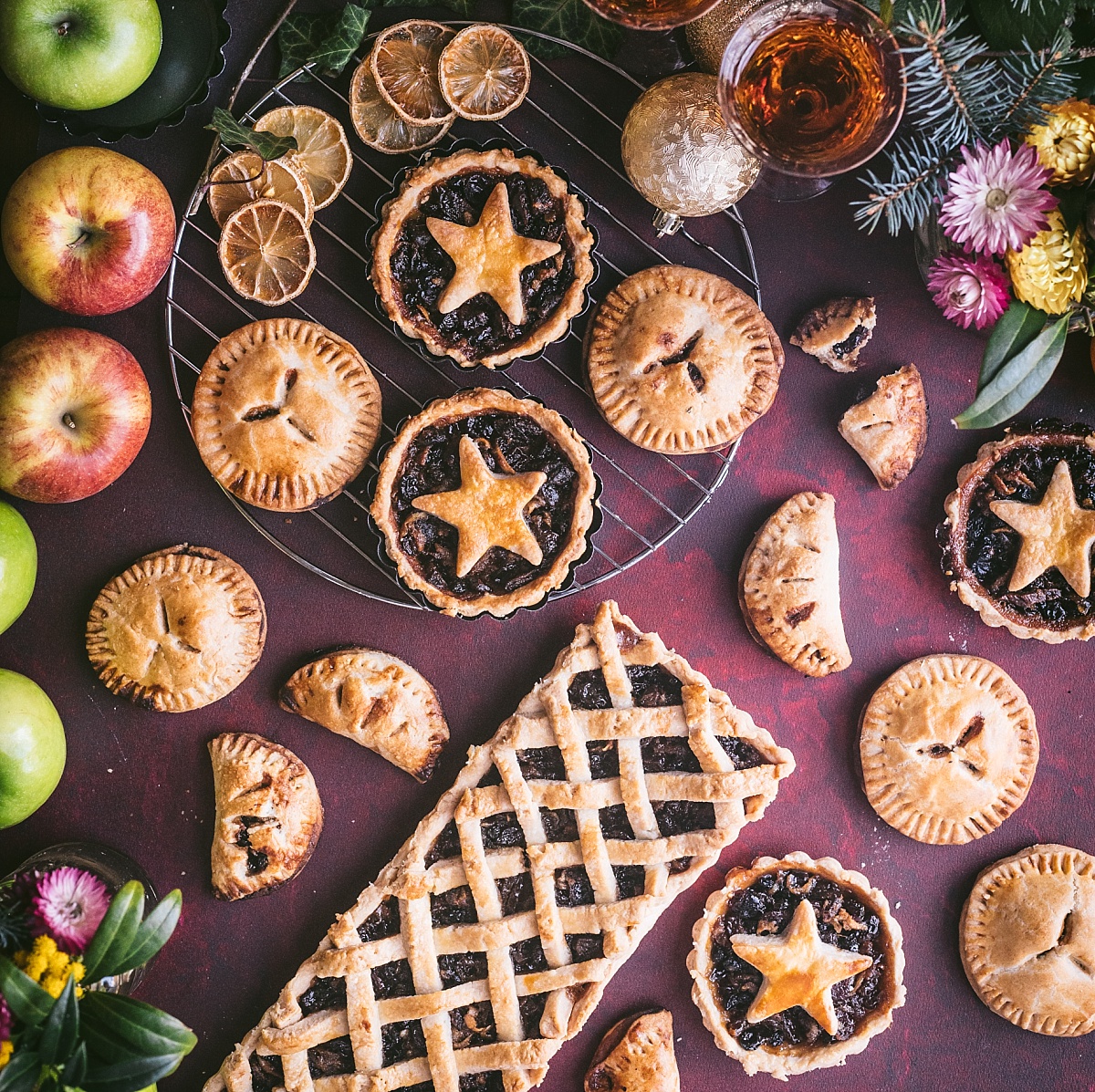This top-down photo, possibly created for a food advertisement or design display, features an assortment of artisanal desserts and fresh apples arranged on a purple and bluish-black background. Focused in the upper right-hand corner are clusters of vibrant purple and yellow flowers, enhanced with green leaves. On the bottom left, additional purple flowers intermingle with leaves and yellow blooms. Dominating the central arrangement are various pies: notably, two small pies with star-shaped crusts filled with blueberries. A larger rectangular pie with an intricate lattice crust lies prominently below. Scattered above are multiple traditional round pies, some fully crusted and others accentuated with dried lemon or apple slices. On the left side of the image, a neat row of apples runs vertically, starting with two green apples followed by two red apples, and then transitioning back to green. Adding a festive touch, the scene includes elements that evoke a holiday ambiance, such as conifer leaves or Christmas ornaments, framing the carefully curated display.